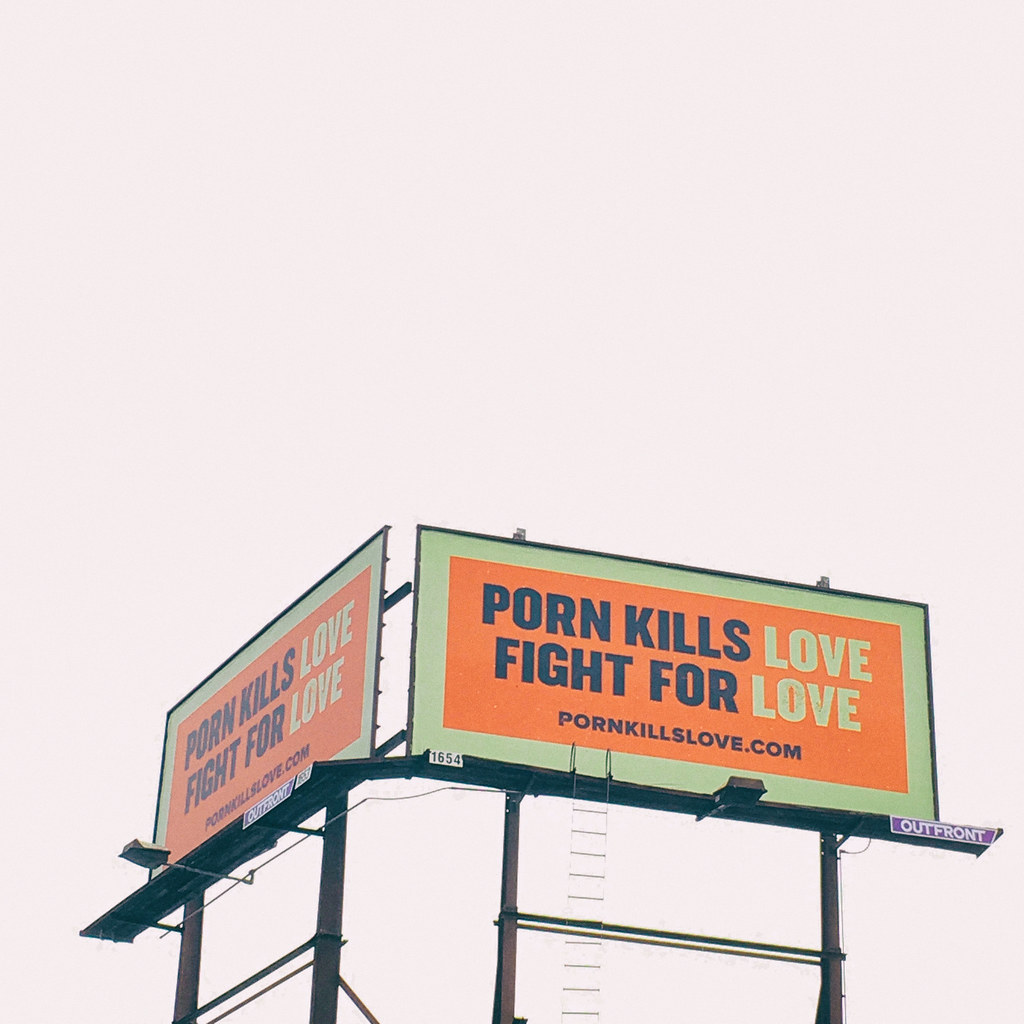The image features three identical billboards set against a gray sky. Two of the billboards face directly forward, while the third is angled to the left. Each billboard is bordered by a thin black frame with a white outline. The main background color of the billboards is orange, with bold black letters declaring "PORN KILLS" at the top, followed by the word "LOVE" in white letters. Below, the message "FIGHT FOR" is written in black, with "LOVE" repeated in white letters beneath it. At the bottom of the billboards, the website "PORNKILLSLOVE.COM" is prominently displayed. The frames of the billboards are equipped with a black ladder for maintenance access. In the bottom right corner of each billboard, a small purple sign states "OUTFRONT" in white letters. Additionally, there is a white sign positioned in the bottom left corner of the image, which features the numbers "1654" in black.